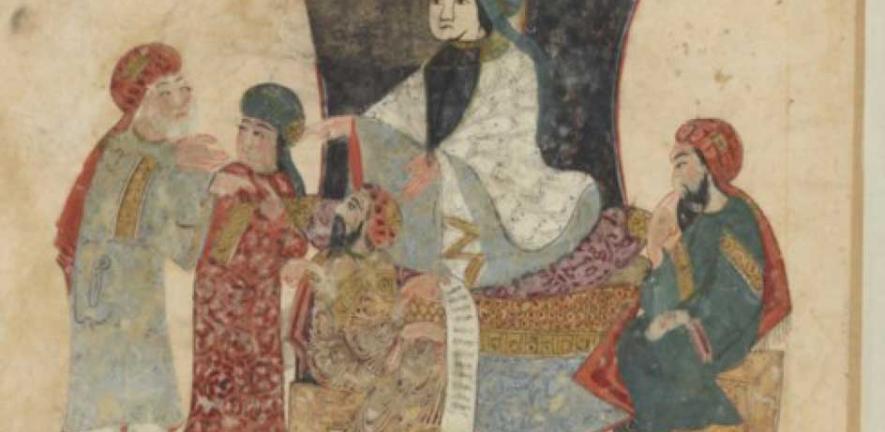This is a color photo depicting an ancient Middle Eastern manuscript or fresco, likely dating back to the 13th or 14th century. The rectangular, horizontal image features a beige-pinkish-off-white background. Central to the composition is a woman seated atop a pile of cushions or possibly a throne, dressed in a white long dress with a black bow, facing to the right. Surrounding her are five individuals dressed in long robes and red turbans with long flowing tails. To her immediate right stands an older gentleman also in a red hat, who appears to be addressing her. In front of this man is a kneeling figure, who seems to be conveying information or paying homage. Positioned to the right side of the frame is another male figure, similarly attired, observing the scene. Each character is drawn with meticulous detail, reminiscent of ancient cultural depictions, suggesting a narrative or a significant moment being captured in this artwork. The collective assembly and their attire indicate a historical context, possibly from the Assyrian or another ancient civilization, emphasizing the importance and ceremonious nature of the gathering.